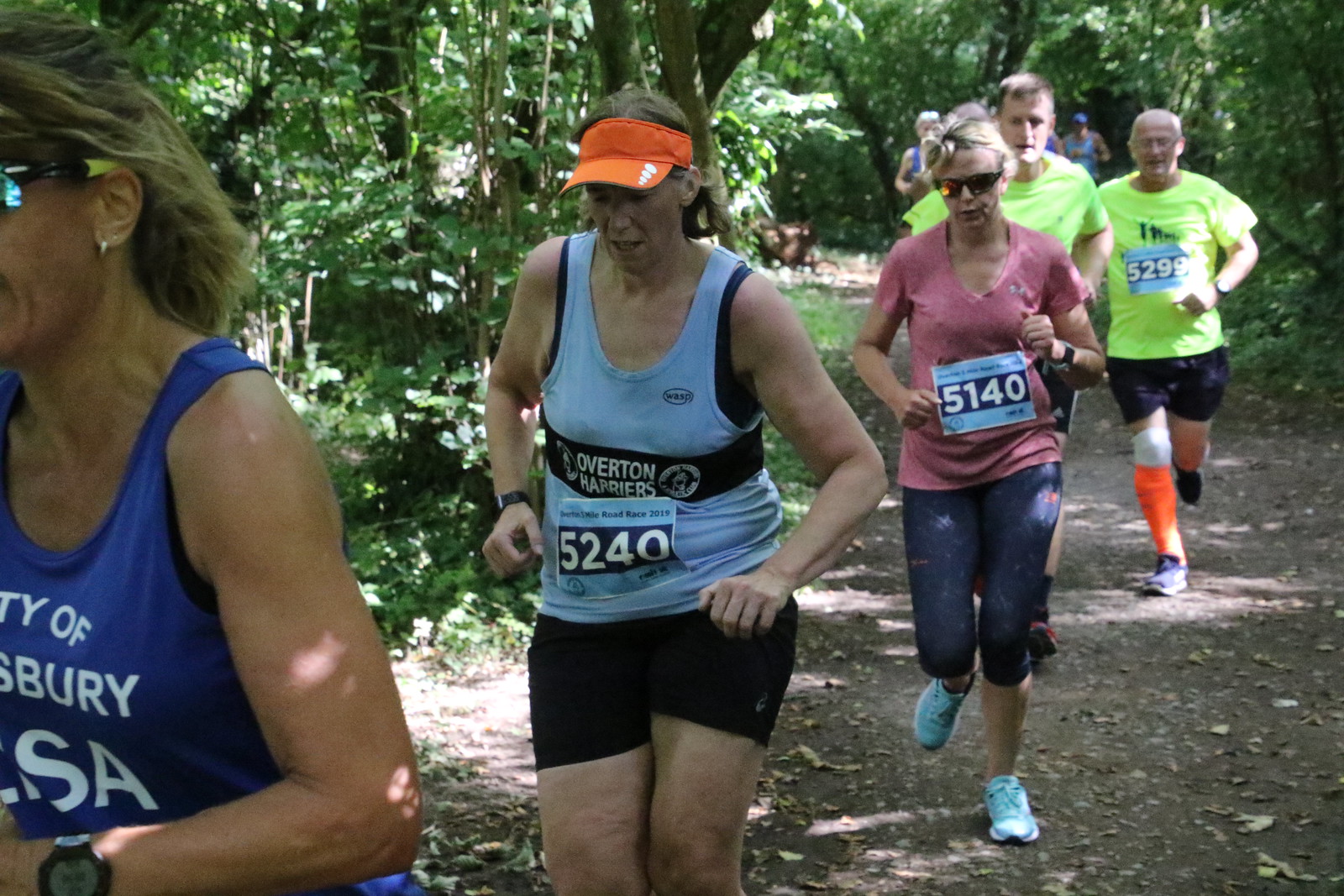In this detailed image, a group of elderly participants, likely over 50 years old, are seen competing in an outdoor marathon on a sunny day. The race takes place on a dirt trail within a forest, where trees with green leaves and brown stems fill the background. The sun filters through the foliage, creating dappled patterns on the ground.

The first runner to the left wears sunglasses and a blue tank top with "City of [illegible] Berry, USA" written in white letters. Her bleached blonde hair with brown highlights is partially cut out of the picture. She also sports a watch on her wrist. Behind her is a woman in an orange visor, wearing a light blue shirt over a darker blue one, coupled with black shorts. Her race number "5240" is displayed on a blue tag with a black background and white text.

Next in line is a woman in a V-neck pink shirt and knee-length black tights, displaying the race number "5140" on a similar tag. Further back, two men wearing highlighter yellow shirts and black or blue shorts are visible, one of whom has an orange leg brace. Their outfits and visible exertion underscore the competitive spirit of this picturesque, forested marathon.